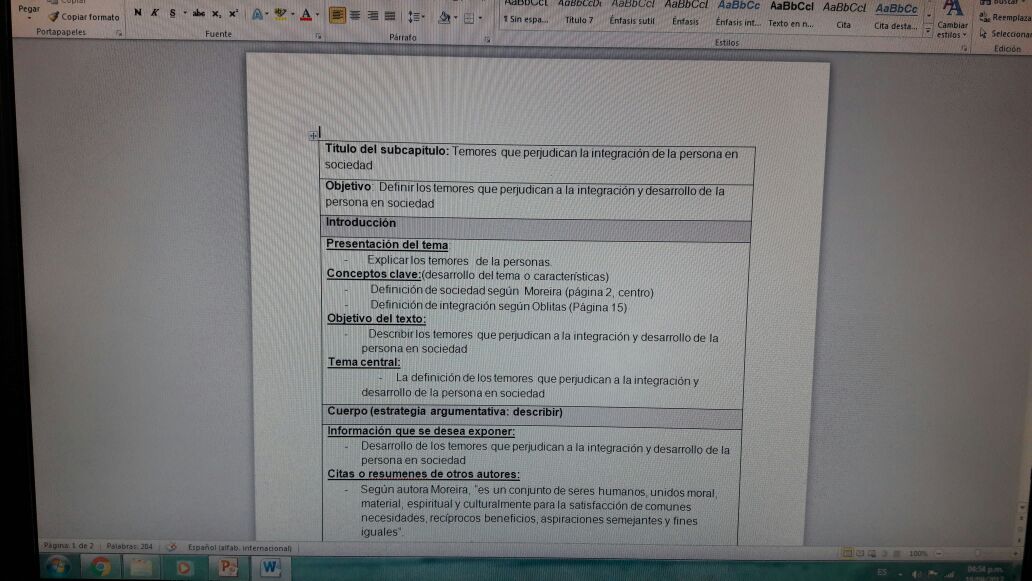The image captures a photograph of a Dell computer monitor displaying a screenshot of a Microsoft Word document. The Dell logo is visible in the bottom left-hand corner, indicating the brand of the computer. The Word document on the screen is formatted in a table/chart layout, entirely in Spanish, with the titles highlighted in gray. The content seems related to a presentation, including sections like "Introduction," "Objectives," and "Concepts." The photograph was taken from a slight distance, revealing typical wavy lines associated with photographing screens rather than capturing digital screenshots. The Windows operating system is visible, with the time shown as 4:54 p.m. Open applications in the taskbar include Microsoft PowerPoint, Google Chrome, and a Microsoft video player.